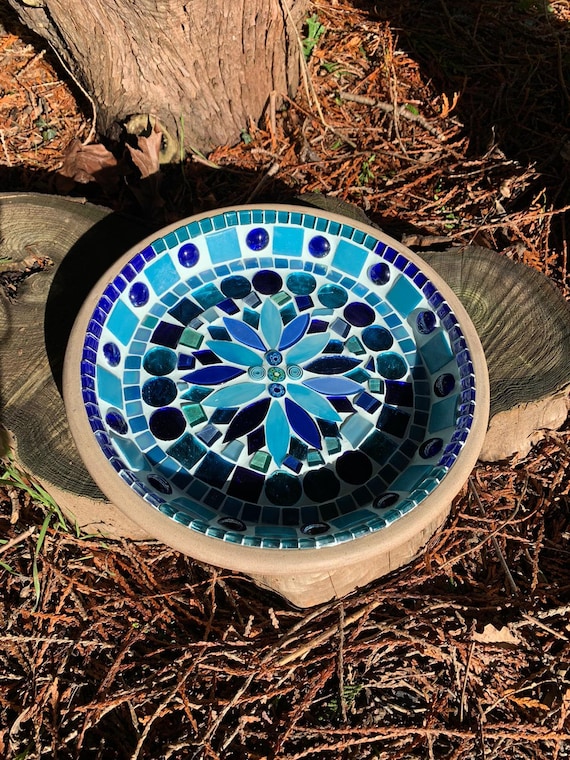The image is a vertical rectangular photograph of a large, round pottery bowl made from brown terracotta clay. The bowl, which features a handle on each side, is placed outdoors on the ground, likely atop a couple of tree stumps. The background is filled with fallen branches and leaves, indicative of a wooded area, with the partial trunk of a large tree visible.

The inside of the bowl is intricately decorated with a glazed mosaic pattern. At the center, there is a motif of blue and green flowers or leaves. Surrounding this are concentric circles of different shades of blue, transitioning through various patterns—diamonds, squares, and circles. These patterns alternate and cascade outward, featuring lighter and darker blue tiles interspersed with white. The edge of the bowl is framed by an additional layer of squares and circles, creating a final, harmonious border. The overall composition and setting suggest a professional photoshoot, showcasing the bowl's elaborate design amidst a natural, textured backdrop.